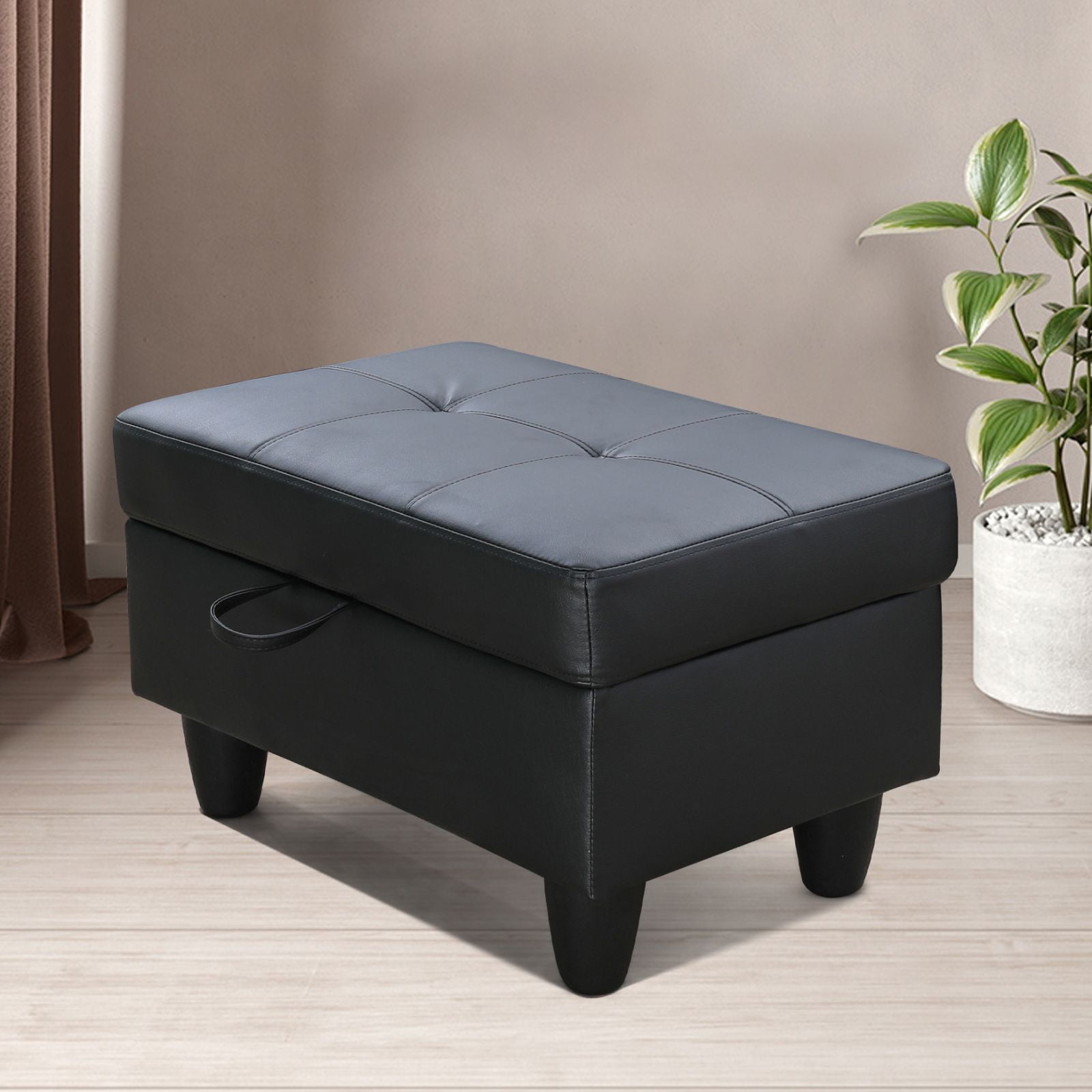In the image, there is a sleek, black rectangular table that appears to double as seating with a cushion on top. The table has four legs, though only three are visible due to the isometric view. The cushion on top suggests it can be used as a footrest or small seat, and on the left side, there's a handle or thread that likely lifts the cushion to reveal storage space underneath. To the right is a vibrant green plant with broad leaves, planted in a grey cylindrical vase filled with pebbles. On the left side of the room, brown curtains allow sunlight to filter in. The room itself has a light grey wooden floor and walls that are a similar shade, creating a neutral and cohesive backdrop for the furniture. The overall decor exudes a minimalist yet functional aesthetic.